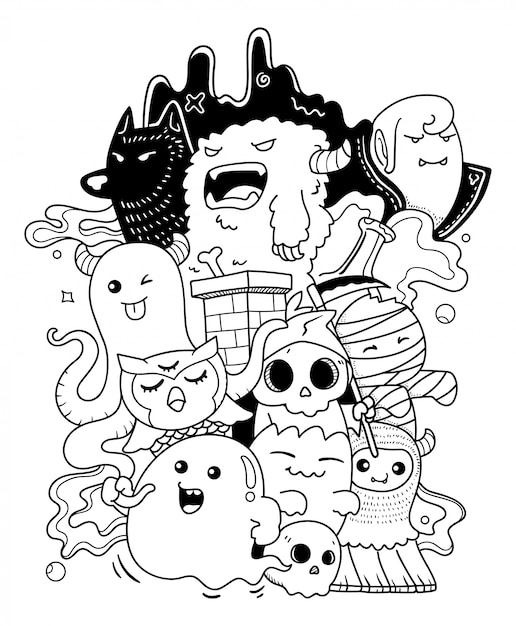This black-and-white illustration, reminiscent of a graphic novel style, depicts a playful yet slightly eerie gathering of Halloween and horror movie characters. The detailed line drawing features a variety of creatures rendered predominantly in black lines against a white background. At the bottom, there's a cute ghost and a charming demon, while higher up, a sweet mummy, an adorable Grim Reaper with a skull face, and a delightful owl make their presence known. Above them, a whimsical octopus with horns and a mischievous gremlin monster add to the collection. Dominating the top left is a darkly shaded werewolf with a stark white nose and eyes, contrasting against its black fur. On the top right, a rotund and endearing Dracula peers out. The illustration is characterized by its solid, intentional lines, with a striking black-shaded area at the top adding depth to the predominantly white composition.